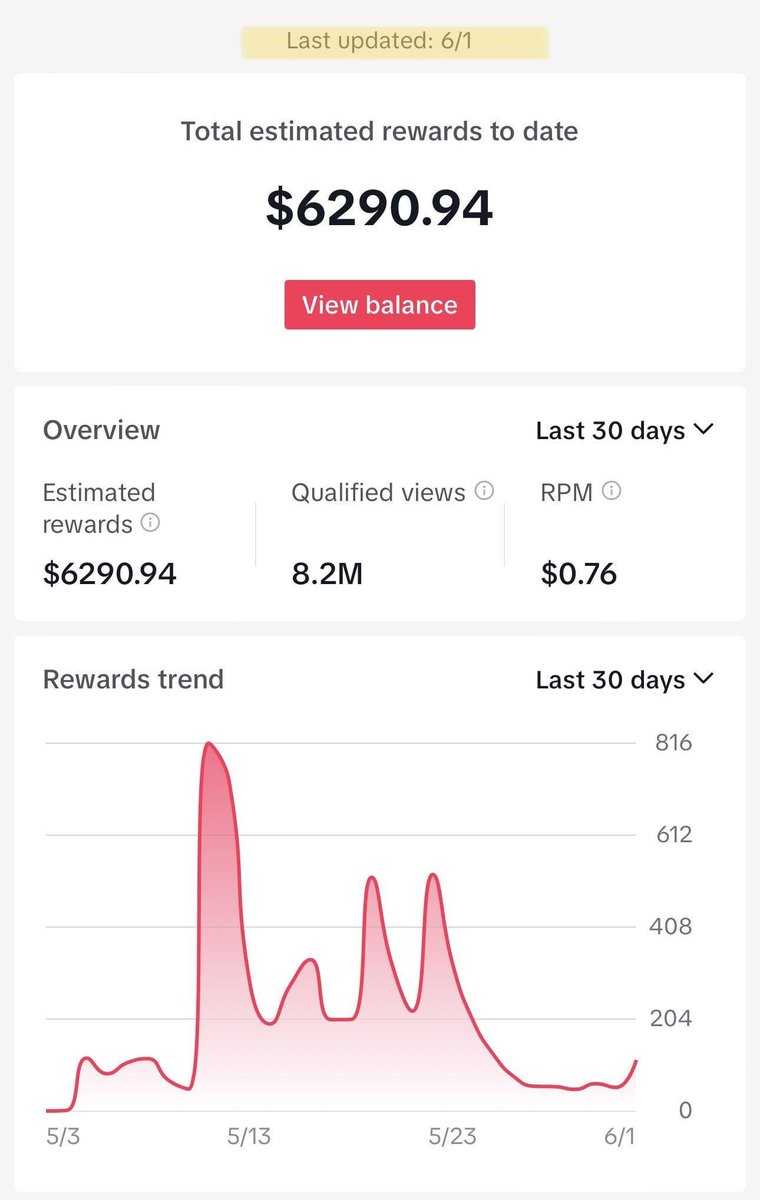This detailed screenshot from a phone features a light gray outline border around the entire box, which is wider at the top. At the center, a smaller yellow rectangle displays "Last updated 6/1." Directly below, a white rectangle centers the text, "Total estimated rewards to date $6,290.94." Beneath this, a red button with "View balance" typed in white invites user interaction.

Further down, another white rectangle appears, divided into two sections. On the left-hand side, it reads "Overview," while the right-hand side displays "Last 30 days" with an adjacent drop-down menu. From left to right, the categories "Estimated rewards," "Qualified views," and "RPM" are listed, each accompanied by an informational circle icon. Below these labels, the values are displayed as $6,290.94, 8.2M, and $0.76 respectively.

The bottom section of the screenshot presents a graph. The top left side of this section is labeled "Rewards trend," with "Last 30 days" and a drop-down arrow on the top right. The graph stretches from $5.23 to 6/1, delineated with vertical scale markers: $0, $2.04, $4.08, $6.12, and $8.16. A red line traces through the graph, indicating the rewards trend over this period.